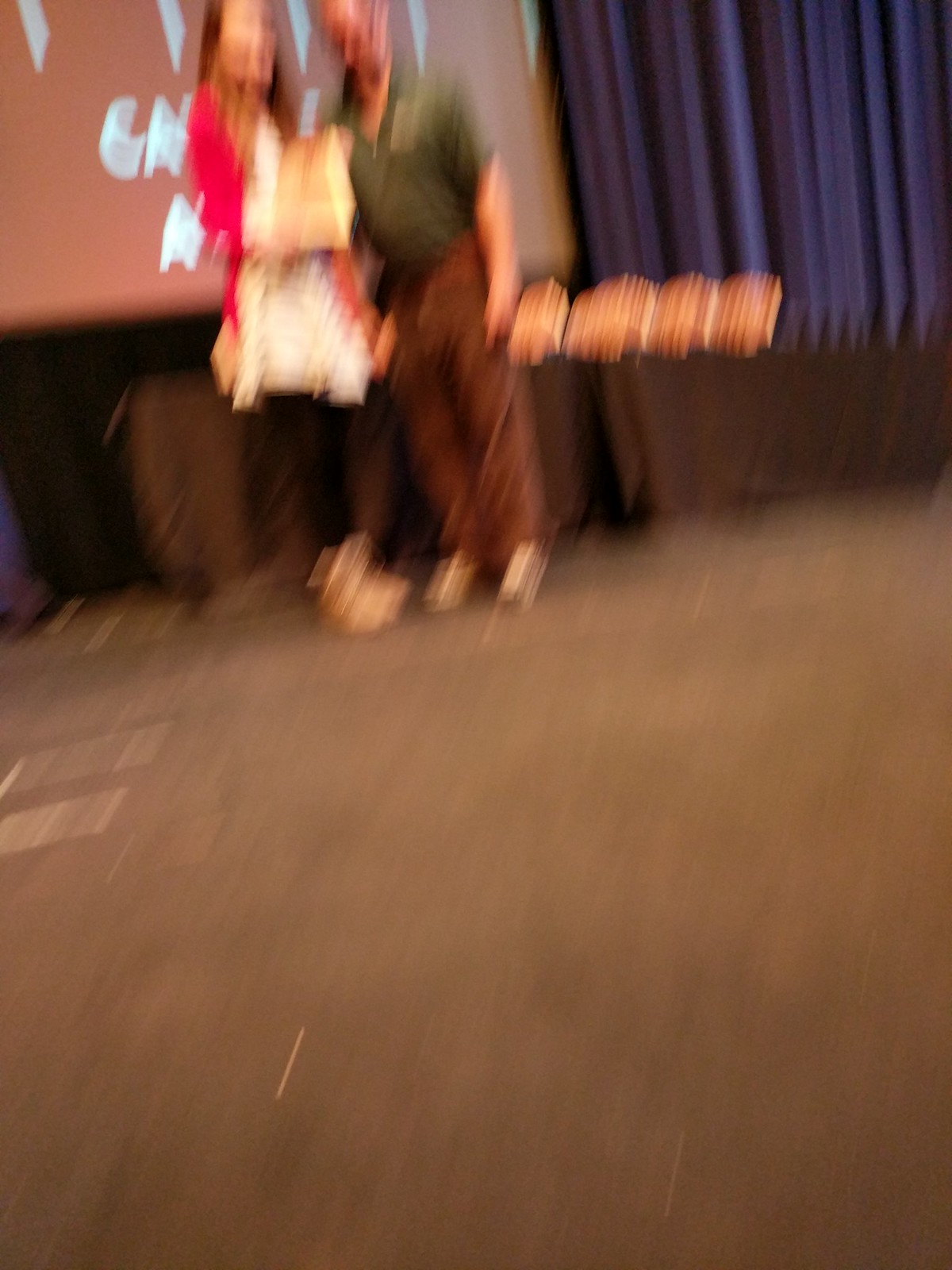This image is an upright rectangular photograph taken indoors, characterized by significant blurriness that suggests the camera was in motion when the picture was taken. The background appears to have brown carpeting, though due to the blur, other shades are also present making it difficult to discern precise details. Blue curtains hang partway down, transitioning to black fabric.

In the center of the image, there seems to be a projection screen displaying a PowerPoint presentation with white text, although the blur makes the content unreadable. In front of the screen stands a man wearing a green shirt, brown pants, and possibly glasses. Beside him is a woman with long brown hair, dressed in a red cardigan over a white tunic paired with black leggings and shoes. The indistinct movement emphasizes that the subjects were relatively stationary despite the overall motion blur.